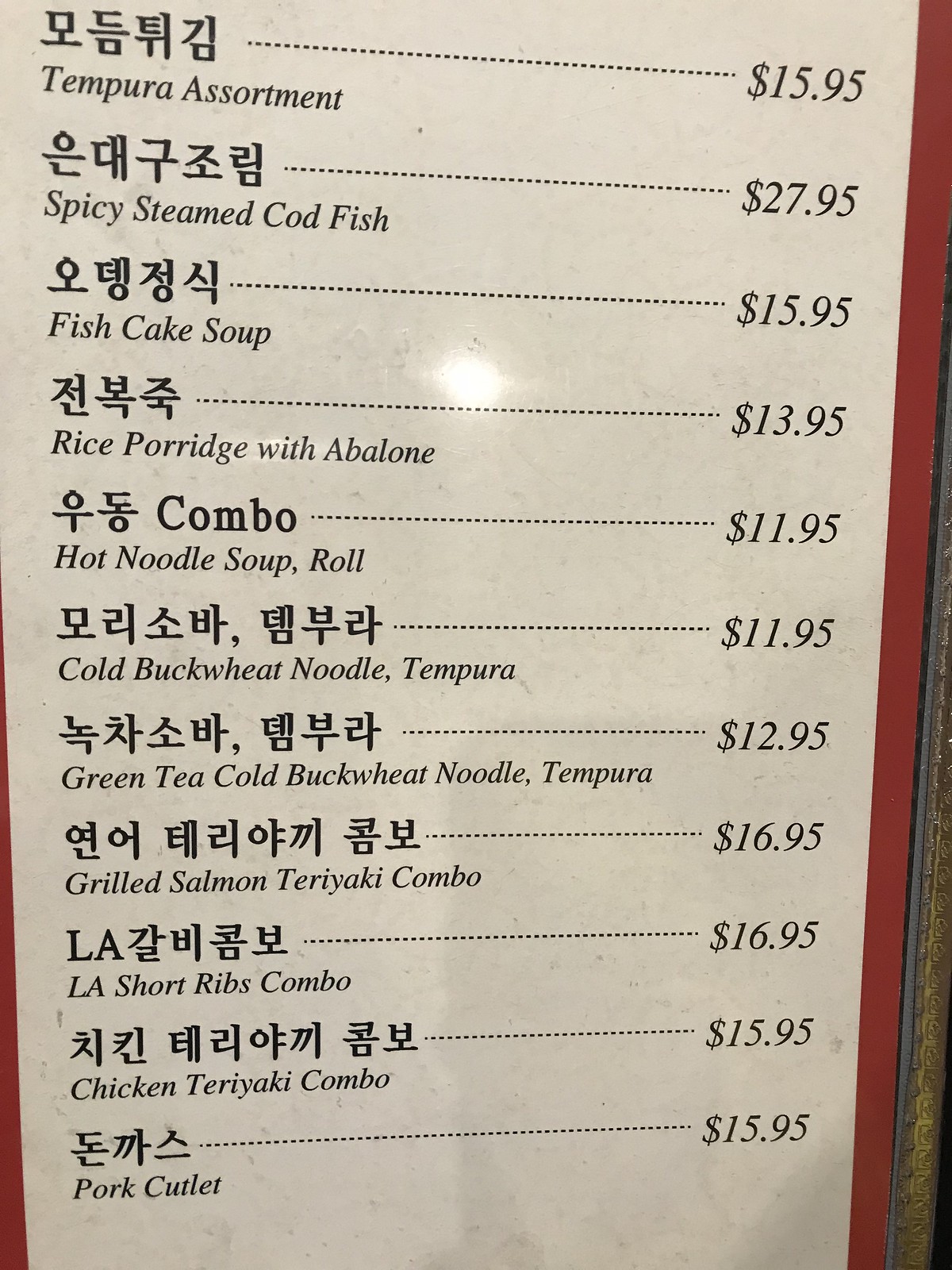The image showcases a restaurant menu that appears to be from an Asian eatery, suggested by the bilingual presentation of dish names in both English and an Asian script resembling Chinese characters. The menu has a clean, white background accentuated by a vivid red border.

At the top of the menu, various selections are listed along with their prices:
1. **Tempura Assortment** - $15.95.
2. **Spicy Steamed Codfish** - $27.95.
3. **Fish Cake Soup** - $15.95.
4. **Rice Porridge with Abalone** - $13.95.
5. **Combo: Hot Noodle Soup & Roll** - $11.95.
6. **Cold Buckwheat Noodle & Tempura** - $11.95.
7. **Green Tea Cold Buckwheat Noodle & Tempura** - $12.95.
8. **Grilled Salmon Teriyaki Combo** - $16.95.
9. **LA Short Ribs Combo** - $16.95.
10. **Chicken Teriyaki Combo** - $15.95.
11. **Pork Cutlet** - $15.95. 

The layout is detailed and structured, making it easy for diners to discern their options while adding an element of cultural authenticity with the inclusion of Asian characters.